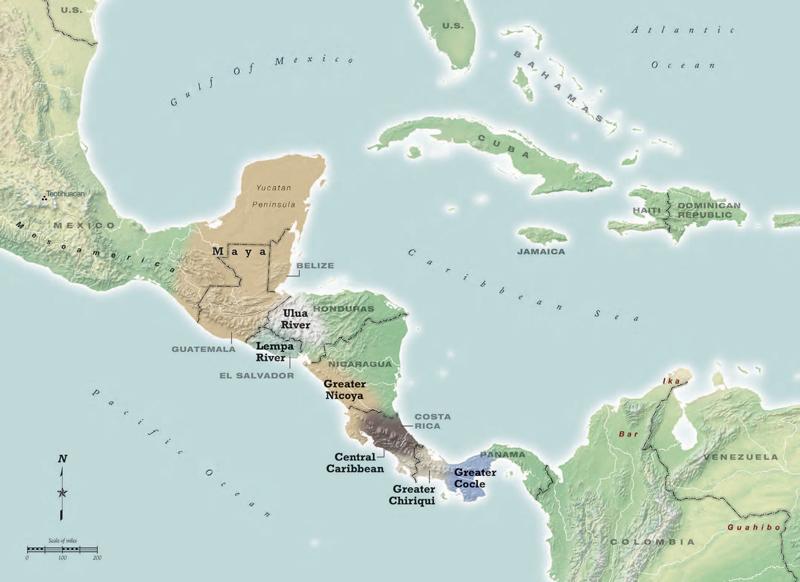This image is a detailed and colorful historical map of Central America and the surrounding regions, illustrated in shades of green, brown, tan, and dark blue. The map includes pre-national divisions and notable geographic features. Key areas depicted are Mexico, the Yucatan Peninsula, the ancient Maya region, the Limpah River, and the Yulo River. It extends to cover present-day countries like Honduras, Nicaragua, Panama, Colombia, and Venezuela. Bodies of water such as the Pacific Ocean, the Caribbean Sea, the Atlantic Ocean, and the Gulf of Mexico are clearly marked. The map also highlights the Bahamas, Cuba, the Dominican Republic, and the tip of Florida, with a small section of Texas visible. Notable regions like the Greater Nicoya, Central Caribbean, and Greater Coquille are labeled. A compass pointing north and a distance scale ranging from 1 to 200 miles enhance the map's utility.